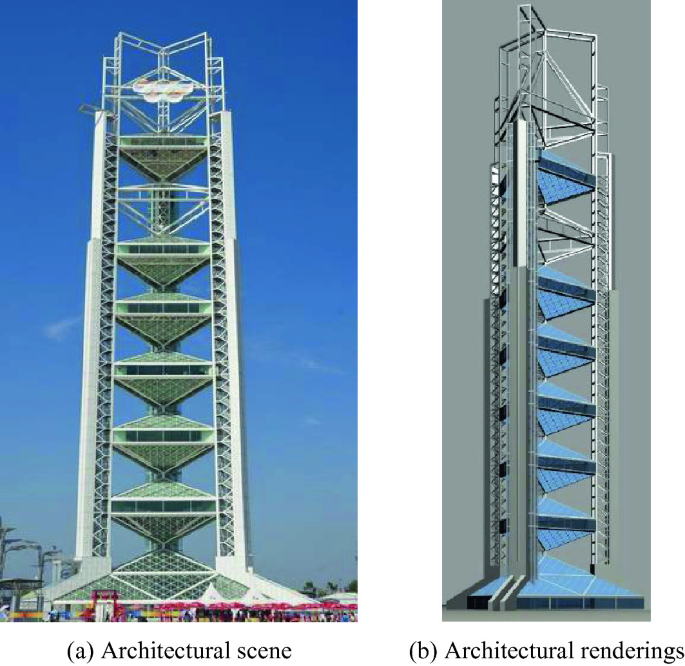This image displays two side-by-side pictures denoted as A and B: an architectural scene (A) on the left and architectural renderings (B) on the right. Both depict a modernistic, tall, cylindrical structure distinguished by its thin, open design. The left photo, titled architectural scene, captures the completed building featuring two main columns with eight diamond-shaped sections running vertically between them. This structure has nine segmented levels, each supported by poles at the top. The right image, labeled architectural renderings, represents the pre-construction sketch of the same structure, also showcasing the segmented center and poles, but facing slightly to the right. The rendering contains triangular blue sections spanning potentially seven stories, while the actual building displays these sections in green. The architectural scene suggests a lively environment at its base, possibly a fair, under a beautiful blue sky. The entire structure is likely supported by steel columns at the corners, underscoring its modernistic and unique design, reminiscent of notable World Fair pavilions.